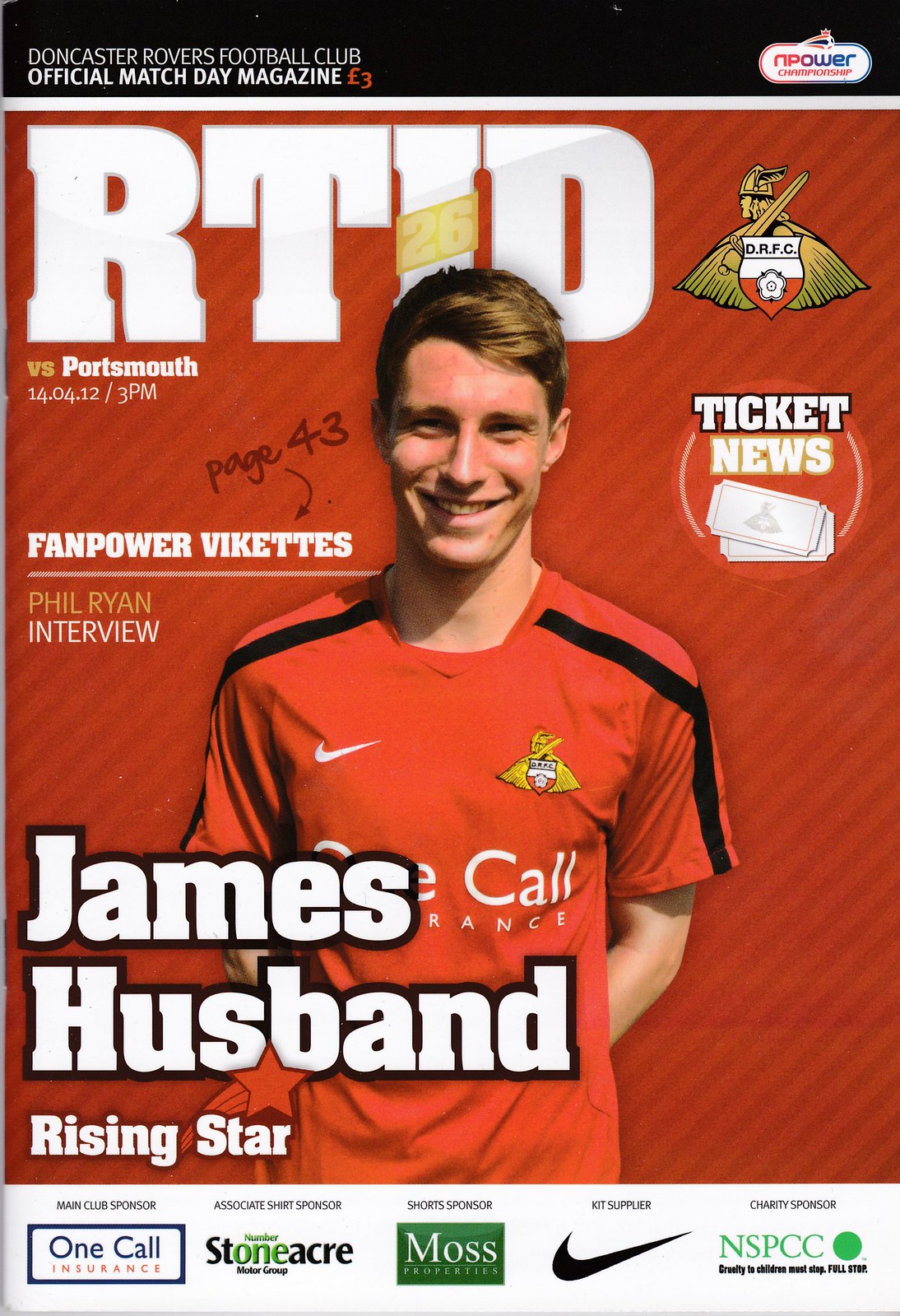The image is a scan of the official match day magazine for Doncaster Rovers Football Club, dated April 14, 2012, at 3 p.m. The cover prominently features James Husband, a young rising star, dressed in a red jersey against a similarly red background. Husband is smiling directly at the camera with his hands behind his back. Large white text in the top left corner reads "R.T.I.D.," and his name, "James Husband," appears in large font at the bottom left corner, accompanied by the label "Rising Star" in slightly smaller text. The magazine has a black border at the top and a white border at the bottom. Additional elements include the Doncaster Rovers FC logo on the right-hand side and text indicating several features like "Fan Power Vaquettes," a "Phil Ryan interview," and "ticket news." Sponsors listed at the bottom include One Call Insurance, Stone Anchor, Moss Properties, Nike, and NSPCC.